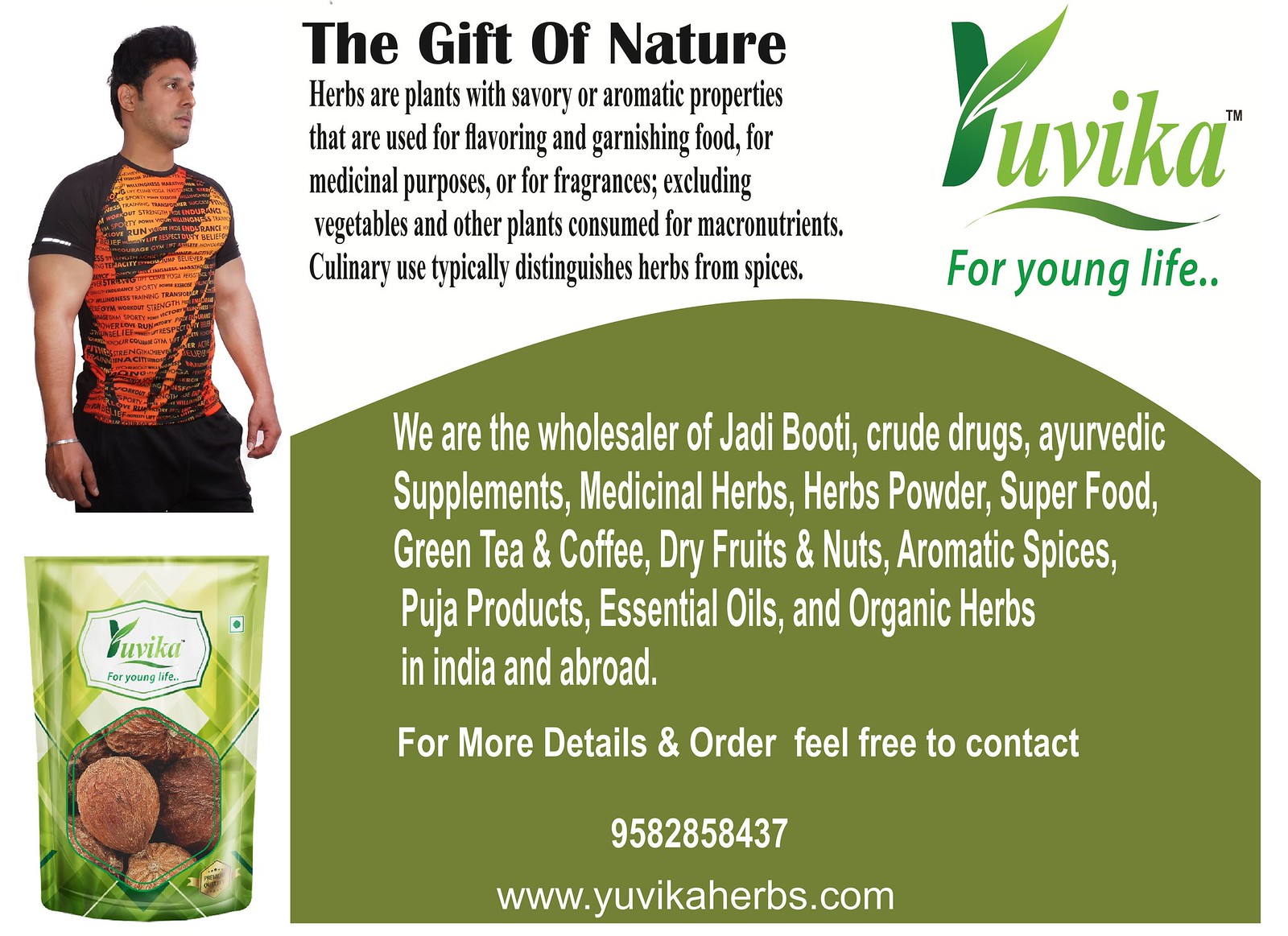The ad is for "Uvica for Young Life" and prominently features the logo where the letter 'Y' transforms into a green leaf amidst a white background. The central tagline "The Gift of Nature" is boldly displayed. Next to it, there is detailed text explaining that herbs are plants with savory or aromatic qualities used for flavoring, garnishing, medicinal purposes, or fragrances, distinct from vegetables and other macronutrient-rich plants, highlighting the culinary differentiation between herbs and spices.

On the right, a muscular male model in an orange and black t-shirt, adorned with motivational words like "Run, Love, Believe," is depicted. He also wears a bracelet on his right wrist and black pants, his gaze directed sideways. Below this image, there is a green rectangular box containing information in white letters: "We are the wholesalers of Jadibhuti, crude drugs, Ayurvedic supplements, medicinal herbs, herb powders, superfoods, green tea and coffee, dry fruits and nuts, aromatic spices, puja products, essential oils, and organic herbs in India and abroad. For more details and orders, feel free to contact 958-285-8437 or visit www.uvicaherbs.com." Adjacent to this, the product itself is showcased in green packaging with various herbs visible inside, emphasizing its premium quality.